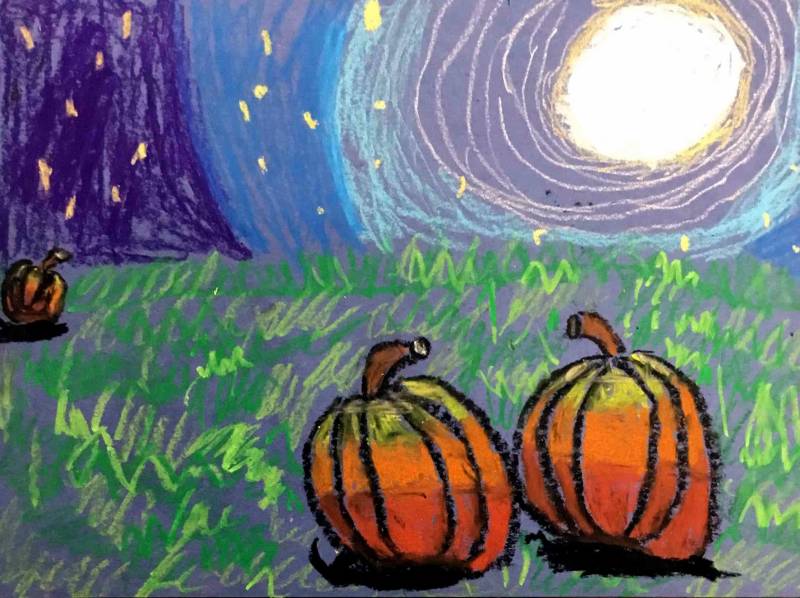The image is a beautifully simplistic crayon drawing of a moonlit pumpkin field. Central to the scene are three pumpkins: two larger ones positioned towards the front, turned slightly towards each other, and a smaller one situated under the base of a large purple tree. The pumpkins, drawn with shades of orange, cast distinct shadows, highlighting the subtle light source from the moon in the top right corner. The sky transitions from dark blue to light blue, featuring scattered white dots that emphasize the night setting. Below, the ground is an array of green tones, depicting grass that has been playfully scribbled across the bottom portion of the image. The primary colors used are green, blue, orange, and purple, making the scene vibrant yet serene, reminiscent of a quiet night in a field under a starlit sky.